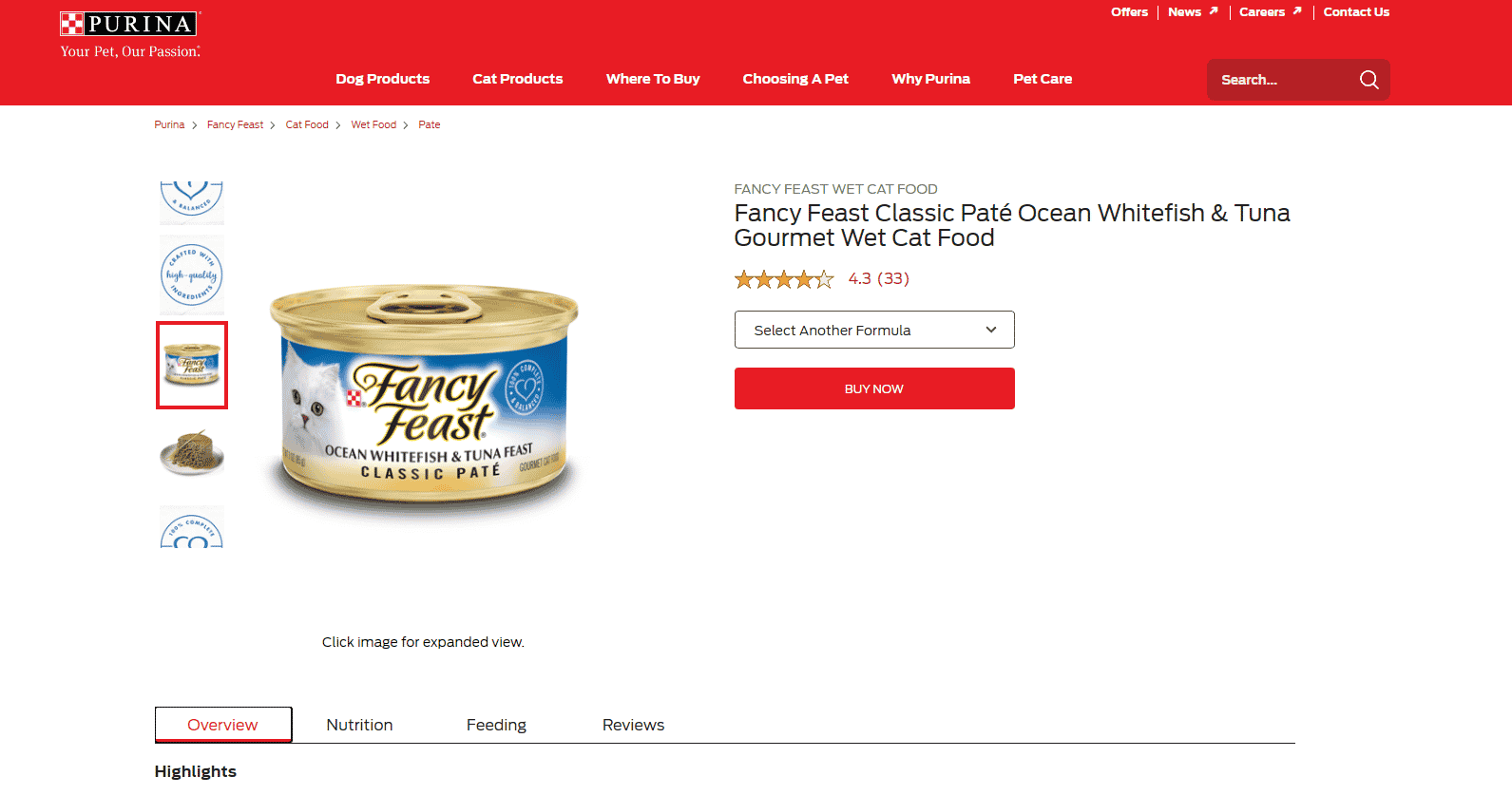**Screenshot of Farina's Website**

The screenshot showcases Farina's website, featuring a dark red band at the top. The top left corner bears the Farina logo: a red square with smaller red squares at the corners, intersected by white squares forming a cross. Attached to this logo is a black rectangle with the bold, white uppercase text "PURINA". Below the logo, the slogan "YOUR PET, OUR PASSION" is displayed in white.

Underneath the logo and slogan, there is a navigation bar with clickable tabs labeled: "DOG PRODUCTS," "CAT PRODUCTS," "WHERE TO BUY," "CHOOSE A PET," "WHY PURINA," and "PET CARE." To the top right, in bold white text, are the links: "OFFERS," "NEWS" (with a right arrow), "CAREERS" (with a right arrow), and "CONTACT US." A search bar in maroon red, with the grey text "SEARCH..." and a grey magnifying glass icon, is also present.

On the left side of the page are multiple images of a specific cat food. One image displays the food outside of the can, appearing as a dark brown and light brown loaf. Another image shows the brass-colored can with bands of blue and white, and a white cat image on the front is highlighted by a red rectangle, indicating its selection. 

A close-up view on the right side shows a white cat with a pink nose looking towards the camera. Next to it, the product name "FANCY FEAST" appears in a cursive black font with a white and gold border. Below this, the Purina symbol is visible, adjoining text that reads "OCEAN WHITE FISH AND TUNA FEAST" in black, and "CLASSIC PÂTÉ" in bold black. The brass-colored can is further detailed on the webpage.

Further down, in all caps and light gray text, it says "FANCY FEAST WHITE CAT FOOD," followed by the regular black text "FANCY FEAST CLASSIC PÂTÉ OCEAN WHITE FISH AND TUNA GOURMET WHITE CAT FOOD." A rating of approximately 4.3 out of 5 stars is displayed, with the stars being gold, except for one partially-filled star. The rating is supported by 33 reviews, indicated by "(33)" in red text. 

Near this section is a drop-down menu with a thin black border, stating "SELECT ANOTHER FORMULA" with a black arrow pointing downwards. Adjacent to this is a clickable burnt orange or red button with the bold white text "BUY NOW." 

Beneath the Fancy Feast can image, it says "CLICK IMAGE FOR EXPANDED VIEW."

At the lower left corner, the "OVERVIEW" tab is selected, featuring red text, a black border, and a red underline. Other tabs include “NUTRITION,” “FEEDING,” and “REVIEWS,” which remain unselected. Lastly, at the bottom left, in bold black text, is the section titled "HIGHLIGHTS."